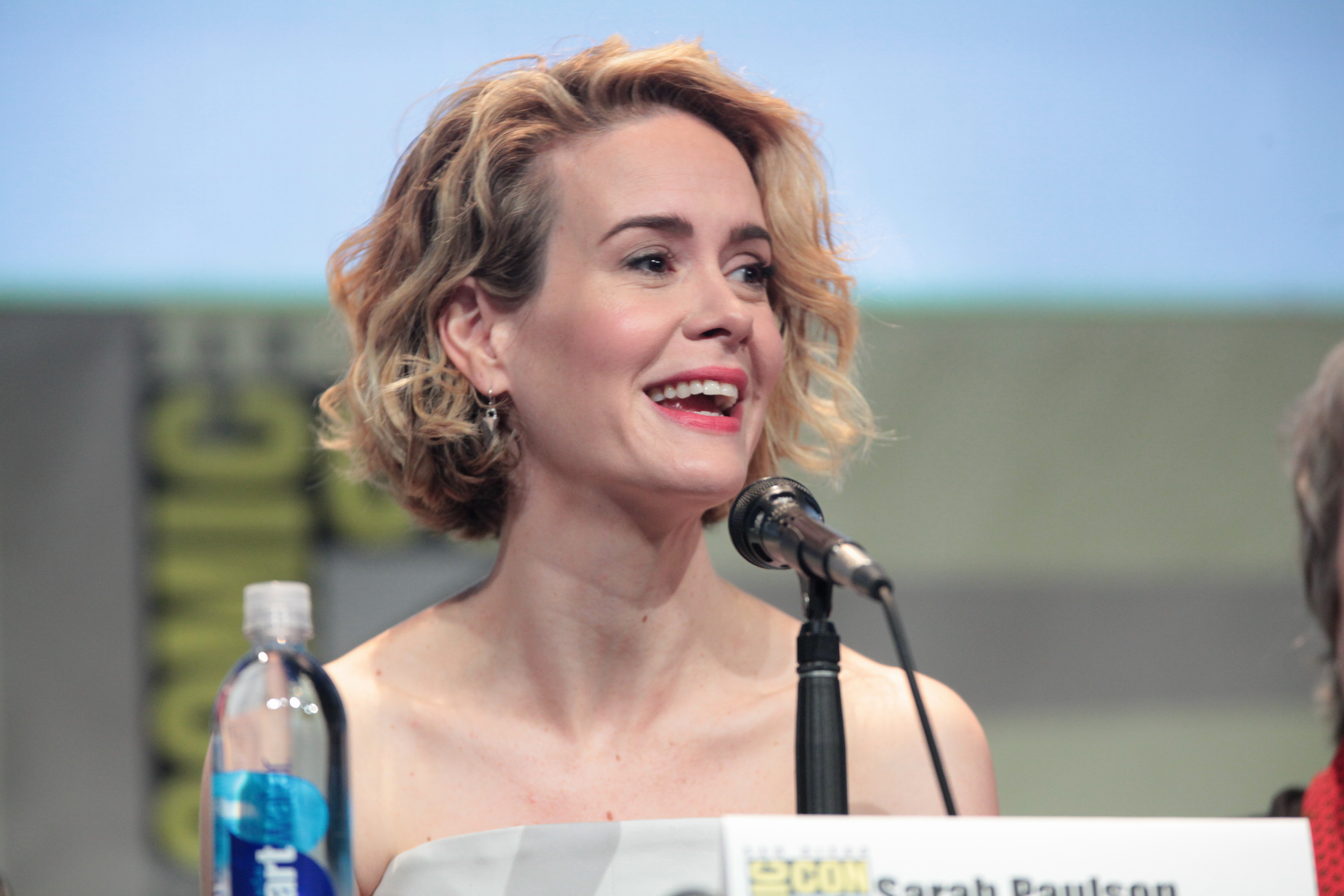The image captures an event at Comic-Con, with a somewhat blurred banner in the background indicating the event's name. Central to the image is actress Sarah Poulsen, recognizable from roles in Marvel films, possibly one of the X-Men movies. Sarah, sporting short, closely-cropped blonde hair, is looking and smiling towards someone off-camera on the right side of the image. She's behind a podium with a microphone and a placard bearing her name. Also visible on the podium is a logo with "Comic-Con" inscribed on it. A bottle of Smartwater is placed to her right (left from the viewer's perspective). The scene is well-lit, with at least three light sources casting minimal shadows, and Sarah appears to be enjoying the interaction at the event.